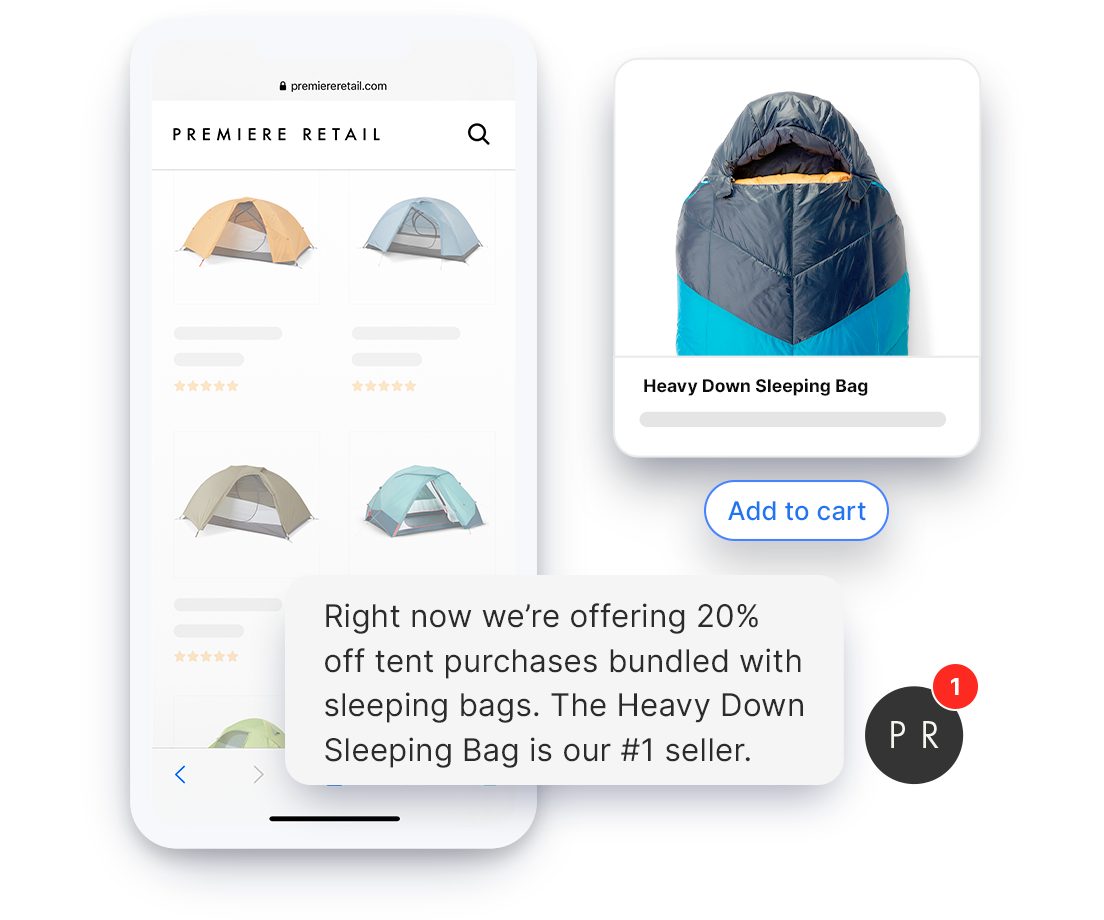The website screenshot showcases "Premiere Retail," prominently displayed in black font on the top left corner next to the ".com" extension. Adjacent to this is the search button. Below the header, a series of vibrant images showcases five pastel-colored tents in pastel orange, pastel blue, pastel brown, pastel greenish blue, and a partially visible pastel green tent. Hovering over these images is a promotional text indicating a 20% discount on tent purchases when bundled with sleeping bags, highlighting the "Heavy Down Sleeping Bag" as the number one seller. 

To the right of the tents, there is an image of the "Heavy Down Sleeping Bag," described in black font. The sleeping bag features a dual-tone design in dark blue and light blue, with a gold-colored center. Below this, there is an "Add to Cart" button. At the bottom of the screen, the "Premiere Retail" logo, featuring the initials "P" and "R," is displayed, alongside a red button indicating that one item has been added to the cart.